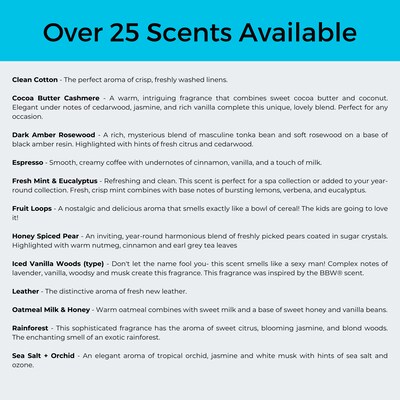The image displays a detailed list of over 25 scents available, with a blue header and black font. Each scent is accompanied by a description. The list includes:

- **Clean Cotton**: The perfect aroma of crisp, freshly washed linens.
- **Cocoa Butter Cashmere**: A warm, intriguing fragrance combining sweet cocoa butter and coconut, with elegant notes of cedarwood, jasmine, and rich vanilla.
- **Dark Amber Rosewood**: A rich, mysterious blend of masculine tonka bean and soft rosewood on a base of black amber resin, highlighted with hints of fresh citrus and cedarwood.
- **Espresso**: Smooth, creamy coffee with undertones of cinnamon, vanilla, and a touch of milk.
- **Fresh Mint and Eucalyptus**: A refreshing and clean scent perfect for a spa collection, combining fresh, crisp mint with base notes of lemon, verbena, and eucalyptus.
- **Fruit Loops**: A nostalgic aroma that smells exactly like a bowl of cereal.
- **Honey Spiced Pear**: An inviting, year-round blend of freshly picked pears coated in sugar crystals, highlighted with warm nutmeg, cinnamon, and Earl Grey tea leaves.
- **Iced Vanilla Woods Type**: A complex fragrance inspired by the BBW scent, featuring notes of lavender, vanilla, woodsy tones, and musk.
- **Leather**: The distinctive aroma of fresh new leather.
- **Oatmeal, Milk, and Honey**: Warm oatmeal combined with sweet milk and a base of honey and vanilla beans.
- **Rainforest**: A sophisticated scent with the aroma of sweet citrus, blooming jasmine, and blonde woods, evoking the enchanting smell of an exotic rainforest.
- **Sea Salt and Orchid**: An elegant aroma of tropical orchid, jasmine, and white musk with hints of sea salt and ozone.

The descriptions offer a vivid sensory experience of each scent, emphasizing their unique qualities and aromas.